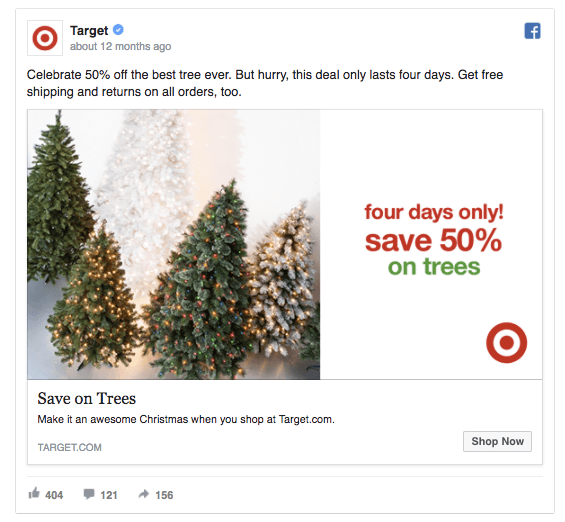Here's a cleaned-up and detailed caption:

---

This is a Facebook ad from Target, posted approximately 12 months ago, announcing a special sale: "50% off the best tree ever!" The offer is valid for four days only, and shoppers can enjoy free shipping and returns on all orders.

The ad features five different artificial Christmas trees, each adorned with various types of lights and decorations. The first tree is white, the second appears to have snow-like decorations, the third tree is unlit, the fourth is small with white lights, and the fifth is taller with multicolored lights.

A text overlay emphasizes, "Four days only: Save 50% on trees." Below it, another line encourages customers to make it an awesome Christmas by shopping at Target.com. The Target website URL is prominently displayed, and the post has garnered 404 likes, 121 comments, and 156 shares. The Target logo is visible twice: once at the top of the ad near the promotional text, and once at the bottom near the call-to-action button that says "Shop Now." A Facebook symbol in the corner indicates that this is indeed an advertisement posted on Facebook.

---

This revision provides a clear and comprehensive description suitable for a marketing caption or advertisement summary.